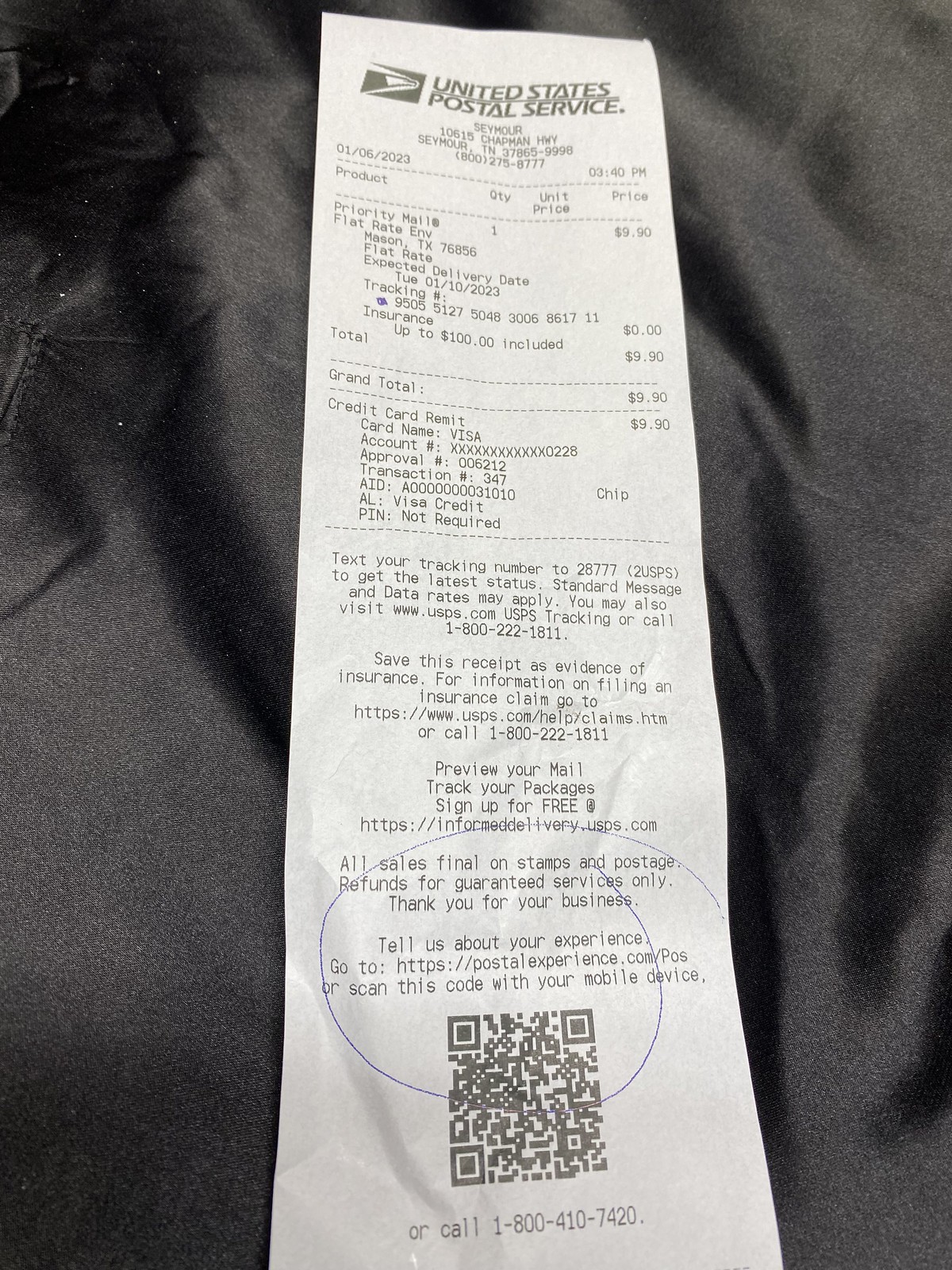A high-quality photograph captures a white receipt with black font, resting on a soft black surface. The receipt prominently features the United States Postal Service logo and the words "United States Postal Service" at the top. Due to a slight glare, the date, which appears to be sometime in 2023, is somewhat difficult to discern. This purchase receipt includes detailed transaction information, including a message that allows customers to text their tracking number to receive updates. The receipt details the purchase total, card issuer information, and contains a circled message at the bottom stating, "All sales are final on stamps and postage. Refunds for guaranteed services only. Thank you for your business." Additionally, it includes an invitation to give feedback about the service, accompanied by a QR code for convenience.